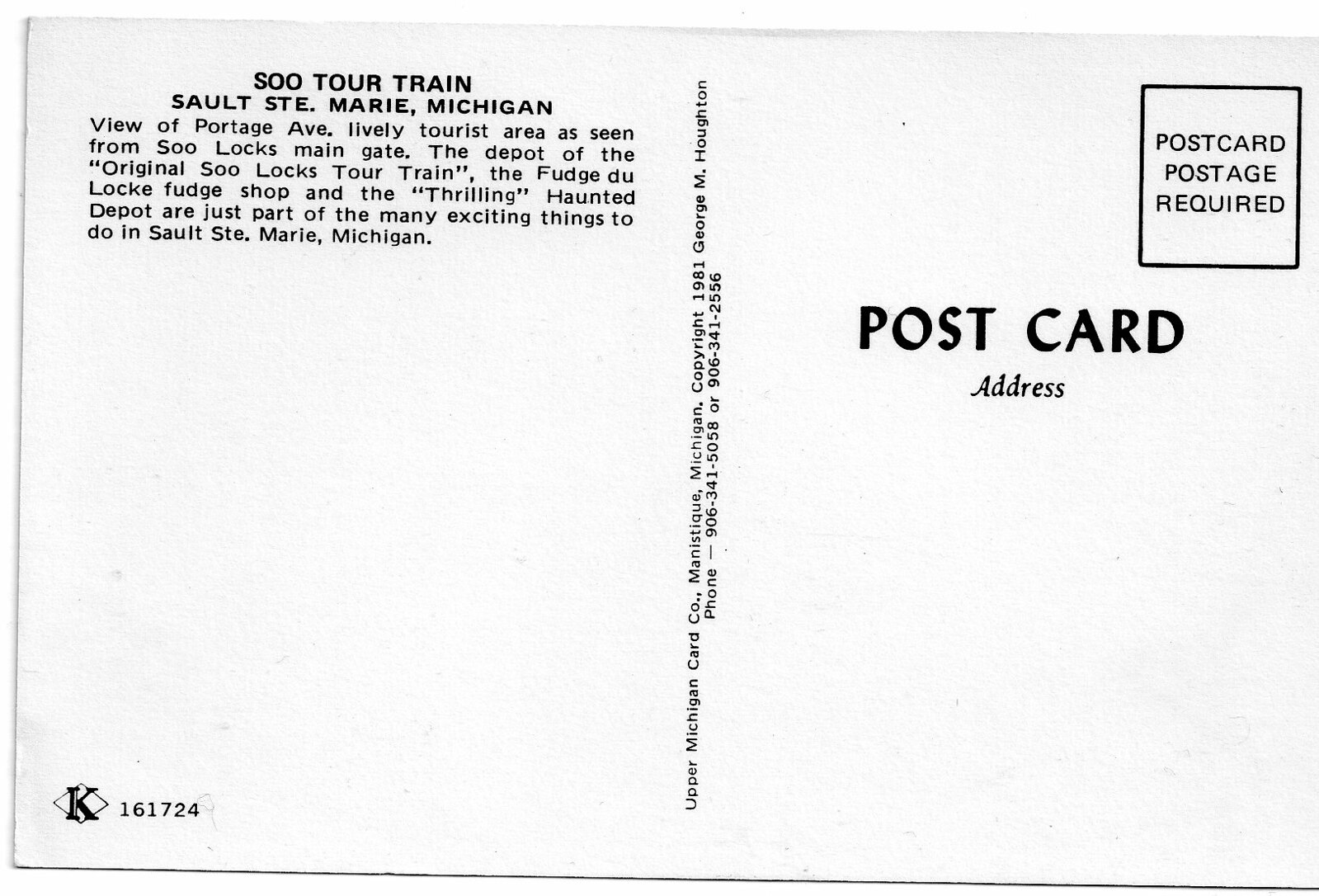The image is a black and white print of the back of a horizontally-oriented postcard. On the left-hand side, the upper-left corner features black print reading "SOO TOUR TRAIN," followed by "Sault Ste. Marie, Michigan." Below that, it describes a "view of Portage Avenue, a lively tourist area as seen from SOO LOCKS MAIN GATE." It mentions attractions like "the depot of the 'original SOO LOCKS TOUR TRAIN,' the 'Fudge DuLock Fudge Shop,' and the 'Thrilling Haunted Depot' as part of the many exciting things to do in Sault Ste. Marie, Michigan." 

The lower-left corner displays a diamond-shaped "K" logo with the number "161724" adjacent to it. Vertically between the left and right sides, it states "Upper Michigan Card Company, Manistique, Michigan, copyright 1981, George M. Hewton," with phone numbers "906-341-505" and "906-341-2556." 

On the right-hand side, the upper section reads "POSTCARD" in bold, dark black, with "address" underneath. The upper-right corner contains a rectangle labeled "POSTCARD POSTAGE REQUIRED." The back of the postcard is divided into two panes, with the left dedicated to descriptive text and the right for the address section.